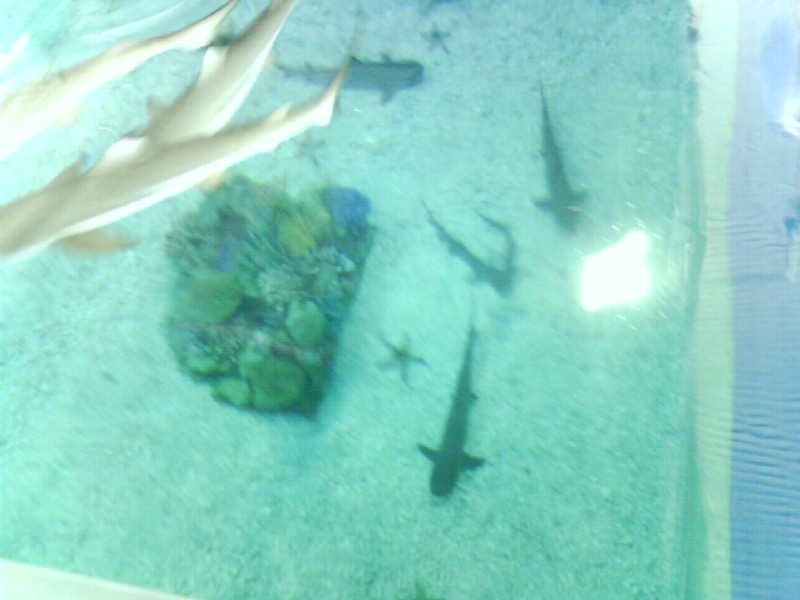The photograph is a vibrant, landscape-oriented color image taken from above, peering into an aquarium tank. The top of the frame features a bright reflection, likely caused by the camera flash bouncing off the glass or perspex surface, which is evident from the non-symmetrical rectangular reflection on the right-hand side adorned with visible scratches. Looking down through the greenish-tinged water, likely a result of light refracting through the aquarium glass, we see the bottom of the tank covered in very small white pebbles. In the center of the tank resides a rectangular block, potentially adorned with coral, surrounded by what appear to be artificial or real aquatic plants. The scene is lively with baby sharks and dogfish swimming about, their numbers ranging around three to four. Most noticeable are the slightly overexposed and blurred sharks near the top-left corner, their heads extending out of the visible frame. Additionally, three dark-colored starfish are scattered on the tank’s base. The lighting, emanating from above, casts a turquoise hue, enhancing the photograph's indoor aquarium setting.